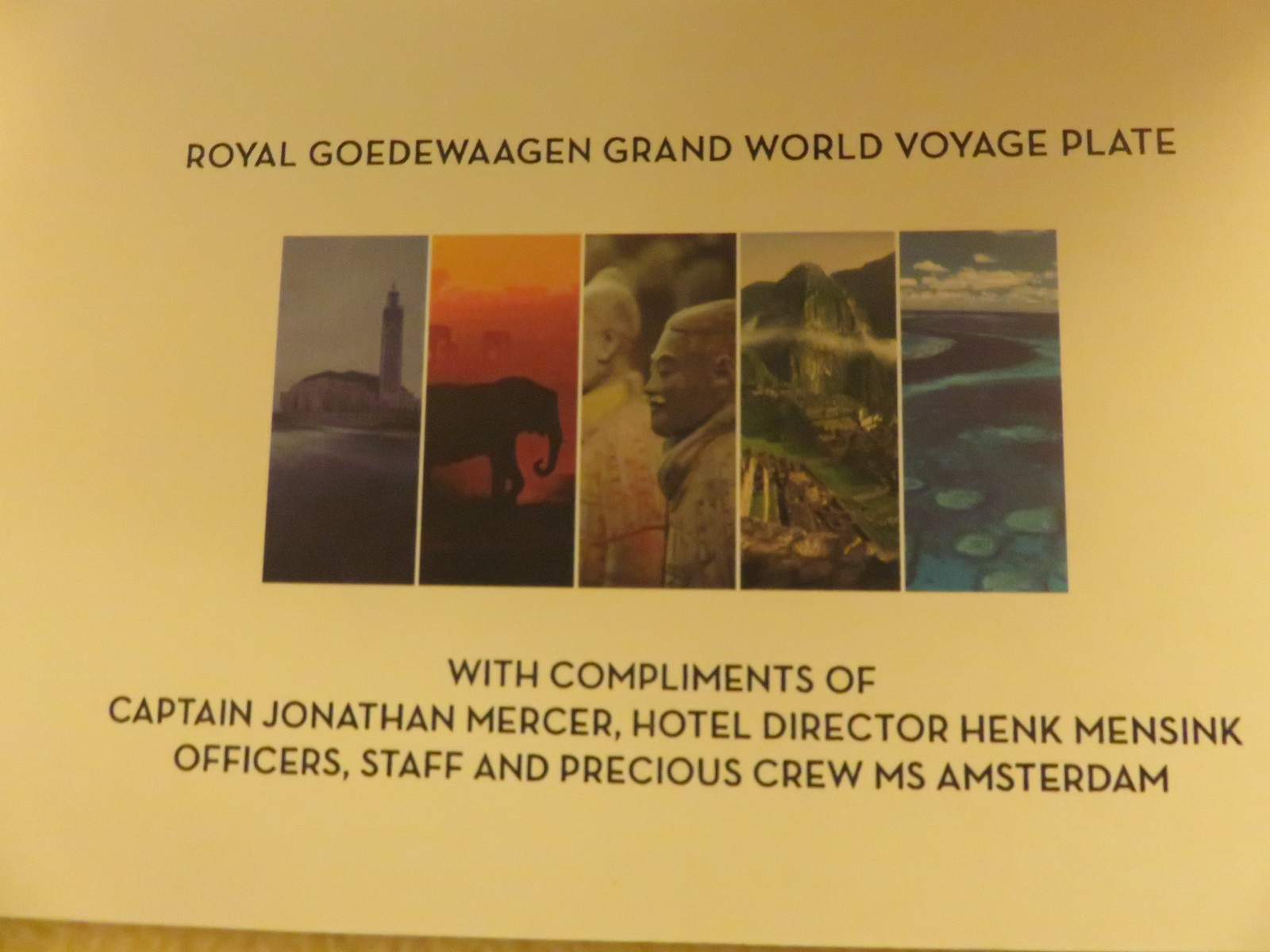A horizontal piece of paper in a yellowish cream color features a series of five narrow, vertical photographs, all aligned side by side. At the top center, in bold black capital letters, the text reads "ROYAL GOEDEWAGEN GRAND WORLD VOYAGE PLATE." The first photograph depicts a distant, misty building that resembles a tower or structure. The second image shows a vibrant orange and red sunset with the silhouette of an elephant standing on grass. The third picture captures an array of Asian statues, reminiscent of the Terracotta Army. The fourth photograph illustrates a hillside featuring brownish rock stairs, possibly alluding to an Incan city like Machu Picchu. The final image presents a serene scene with a blue sky above and greenish-blue water below, suggesting a coastal or beach setting. Beneath these images, the text in black capital letters conveys a warm message: "WITH COMPLIMENTS OF CAPTAIN JONATHAN MERCER, HOTEL DIRECTOR HENK MENSINK, OFFICERS, STAFF AND PRECIOUS CREW, MS AMSTERDAM."